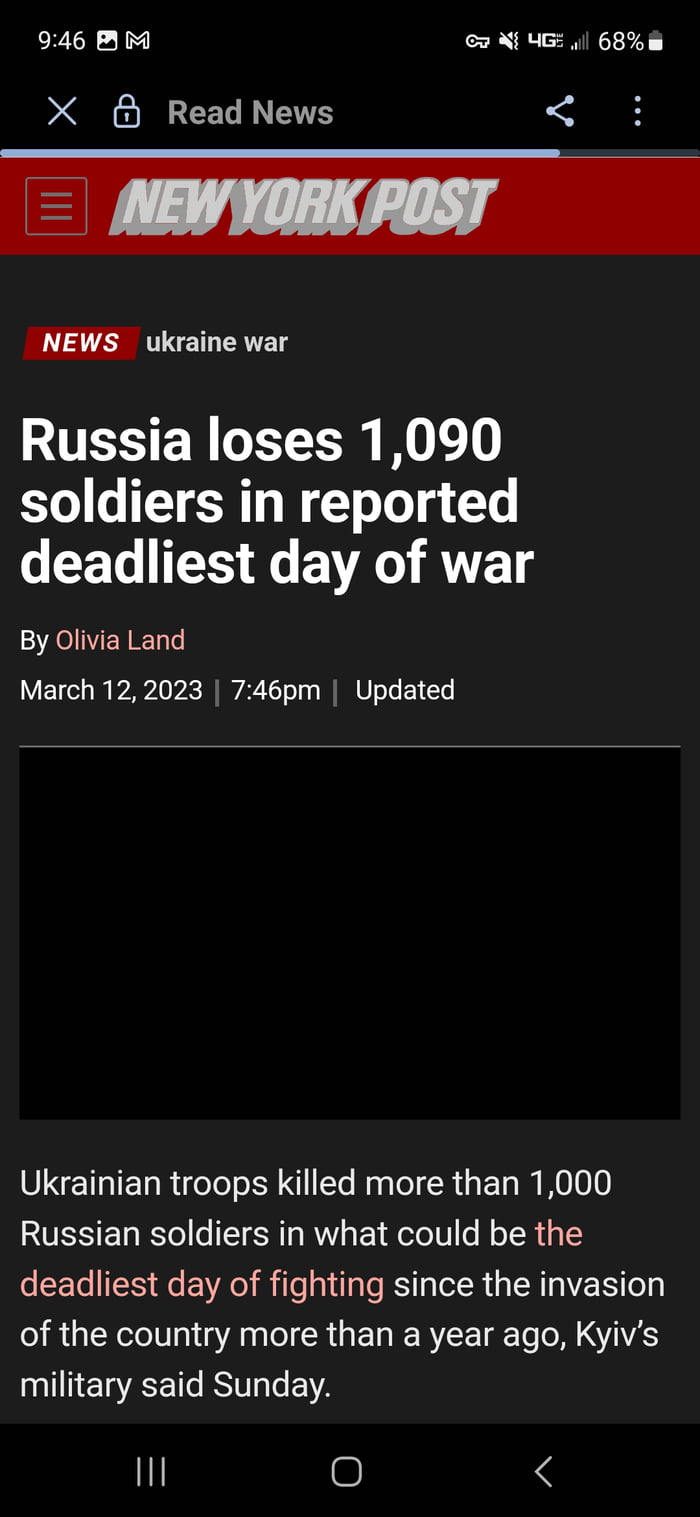This is a detailed screenshot from a person's cell phone displaying a news article. At the top left corner, the time is shown as 9:46, along with icons for "Screenshot" and "Gmail." The top right corner features a white key icon, a speaker icon with a wavy line indicating the phone is on vibrate mode, a 4G LTE symbol, signal coverage bars, and a battery life indicator at 68%. The top banner reads "Read News" with a red header below it stating "New York Post." 

The body of the content starts with "News, Ukraine War. Russia loses 1,090 soldiers in reported deadliest day of war by Olivia Land, March 12th, 2023, 7:46 PM updated." The article reports that Ukrainian troops have killed more than 1,000 Russian soldiers in what is potentially the deadliest day since the invasion began over a year ago, according to Kiev's military. The phrase "the deadliest day of fighting" is accentuated in red letters while the rest of the text is in white. 

The image is purely textual with no photographic, human, animal, avian, plant, or vehicular elements. It is vertically oriented, being taller than it is wide.